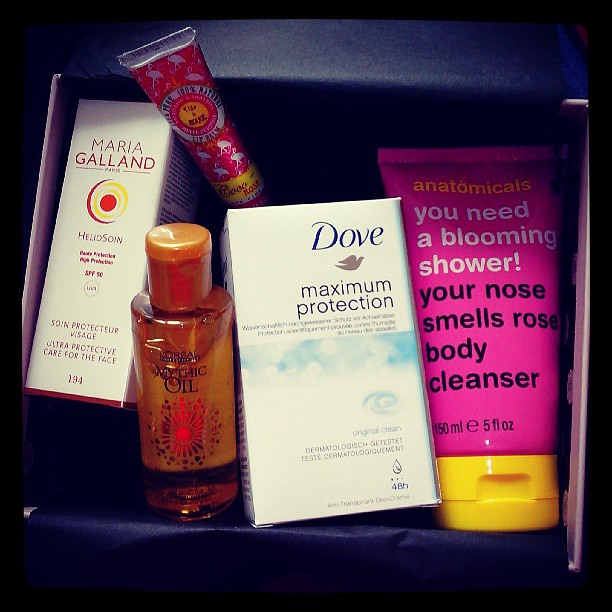The image depicts an open blue gift box with white edges, containing an assortment of beauty products. On the far left, there is a white box labeled "Maria Galland Paris Helio Soyne SPF 50 sunscreen" with a logo featuring a red dot encircled by yellow and red. Adjacent to this is a bottle of L'Oreal Mythic Oil, distinguished by its orange color and matching lid. Positioned above is a lip balm in a grey tube decorated with pink and silver flamingos. In the center of the box is a white box labeled "Dove Maximum Protection Original Clean" with a dove logo beneath. On the right side of the box is a large pink squeeze tube with a yellow cap, branded as "Anatomicals" with the product name "You Need a Blooming Shower, Your Nose Smells Rose Body Cleanser."